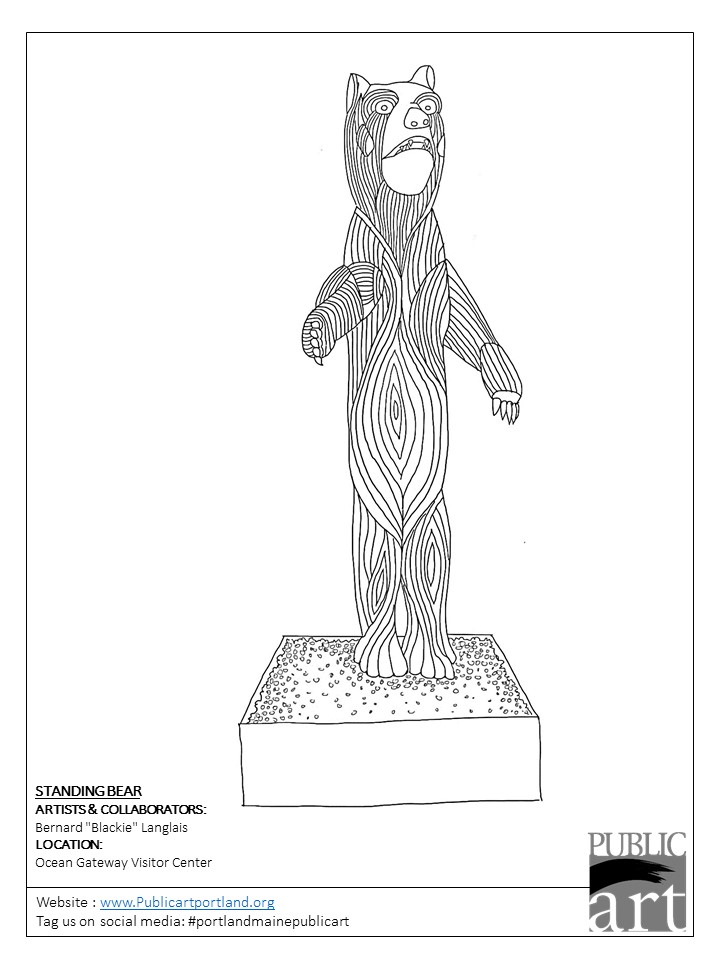This detailed illustration showcases "Standing Bear," a monochromatic drawing by artists and collaborators Bernard "Blackie" Langlais, intended for exhibition at the Ocean Gateway Visitor Center. Rendered in precise black lines against a stark white background, the artwork depicts a slender bear standing upright on a platform, reminiscent of a totem pole and drawn with a pencil-like finesse. In the bottom left corner, clear black text identifies the piece: "Standing Bear," with accompanying information about the artists, location, and the website www.publicartportland.org. The viewer is also encouraged to tag social media posts with #PortlandMainePublicArt. A gray and black "Public Art" logo is positioned in the bottom right corner, encapsulated in a square.